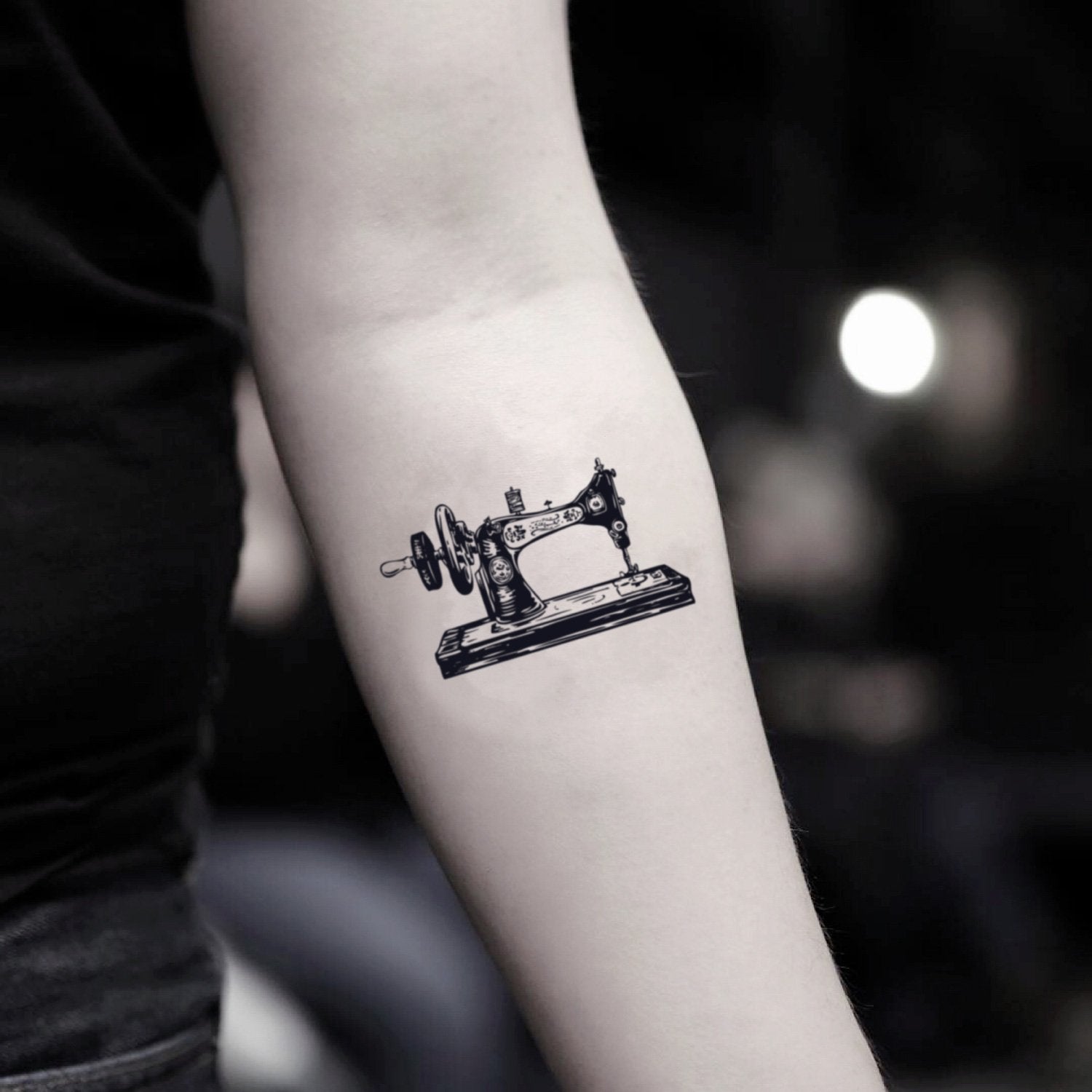This square, black-and-white photograph prominently features the inner part of a young person’s left arm, extending from the crook of the elbow down towards the wrist. The light-skinned individual is sporting an intricately detailed black ink tattoo of an old-fashioned Singer sewing machine, complete with metal components and a manual crank, reminiscent of one of the earliest models. The focal point of the image is the tattoo, set against the person's taut, youthful skin. The individual, who may be female and appears to be Caucasian, is clad in a black shirt and black jeans. In the background, a muted, dark tone with a bokeh effect highlights a small, circular light spot to the right of the elbow, bringing subtle emphasis to the tattoo and the central section of the arm.